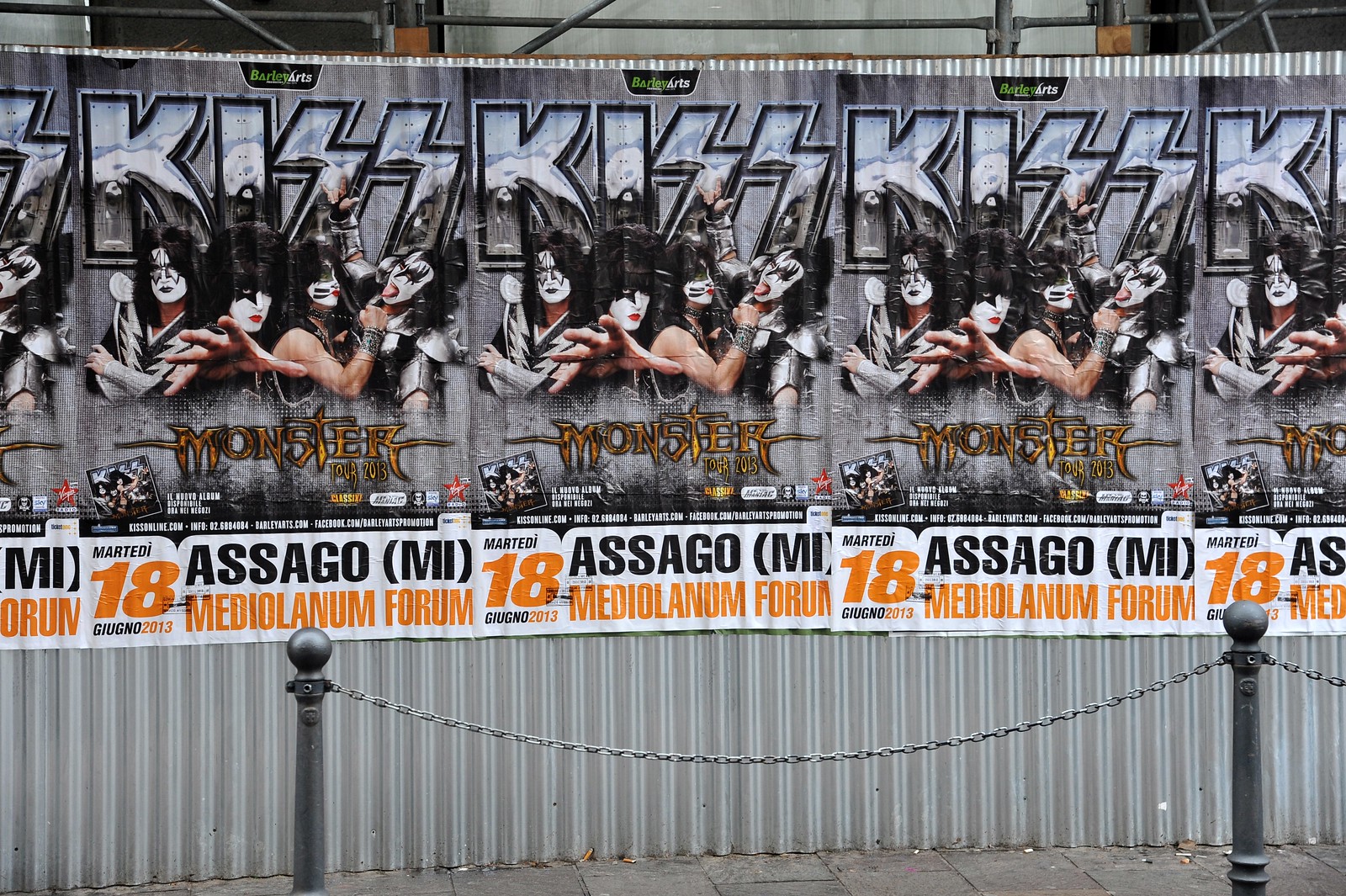The image features a series of five identical posters advertising a concert by the rock band KISS, displayed on a large gray wall with white vertical stripes. The posters are lined up next to each other, with three fully visible in the center and two partially cut off on either side. Each poster prominently displays "KISS" at the top, with the 'S's styled as lightning bolts. Below the band name, the poster features images of the four band members in various poses. Additional text includes "Monster" and the date "18th, 2013." There are also inscriptions reading "ASSAGO" and "MEDIO LANUM FORUM" in black and yellow text, respectively. In the foreground, a black chain-link fence is attached to two black posts, suggesting a roped-off area likely intended for queueing. At the very bottom of the image, a small portion of a sidewalk is visible.